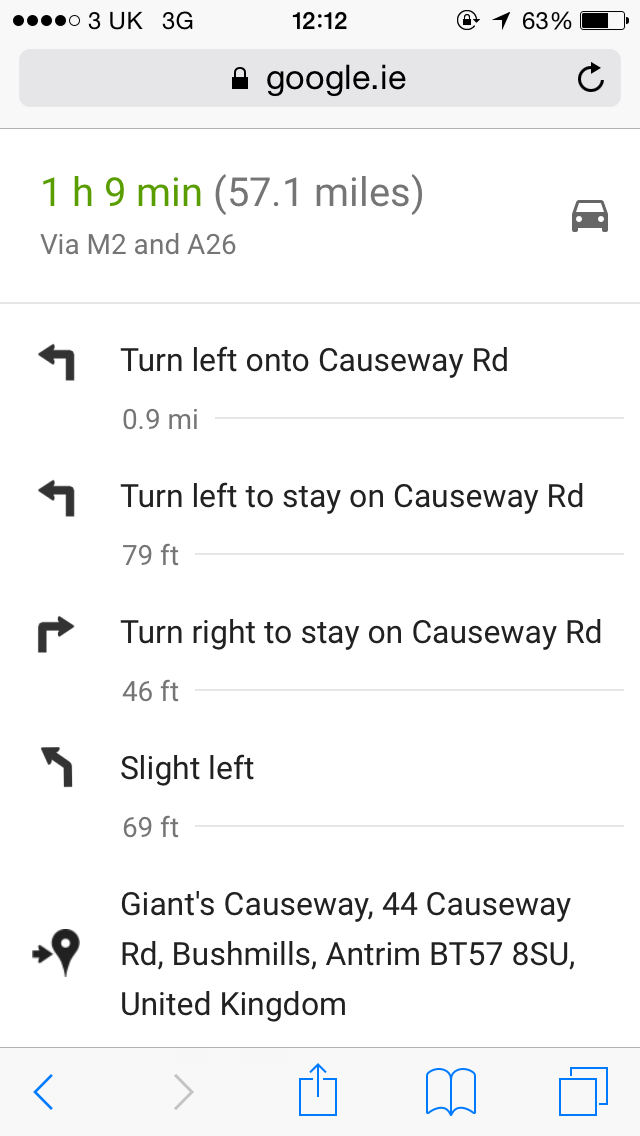This screenshot, likely taken from an Apple device such as an iPad, captures various on-screen details. The status bar at the top shows four bars of cellular signal under "3 UK 3G," with the time noted as 12:12 PM. The device is locked, restricting slide actions, and location services are active. The battery level stands at 63%. This appears to be a screenshot from the Safari browser, with the URL "Google.ie" displayed. It features a navigation route for a destination, suggesting a journey duration of 1 hour and 9 minutes, covering 57.1 miles via the M2 and A26 roads. The instructions detail several turns on Caseway Road, eventually leading to "44 Caseway Road, Bushmills, Antrim, BT57 8SU, United Kingdom," near the Giant's Causeway.